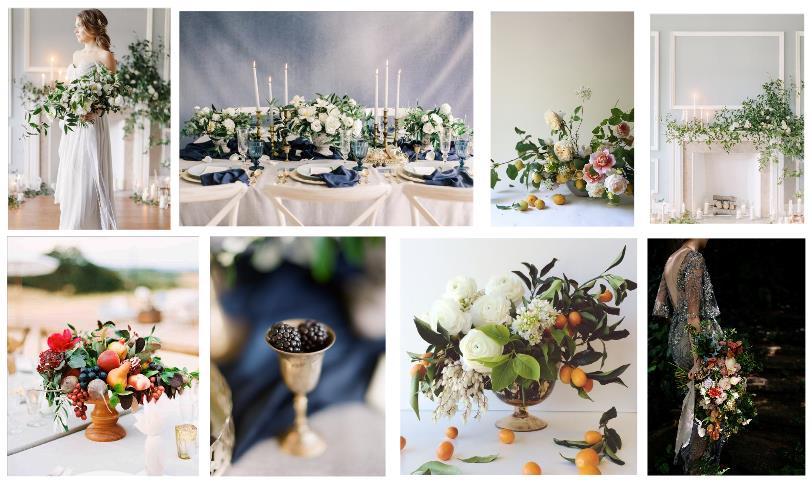This detailed collage features eight images organized into two rows, each row containing four photographs, and primarily depicts a wedding theme with predominant colors of white and green. In the top left image, a bride stands in a white dress, holding a bouquet of flowers with some greenery beside her. To her right, the next image showcases a fully laid-out table adorned with a set of three candlesticks. The centerpiece consists of a larger bowl of white flowers flanked by two smaller bowls, all situated on white plates accompanied by blue napkins. The third image in the top row is a close-up of additional white and pink flowers. The top right image displays a white-painted fireplace with a white candle and some greenery on the mantle.

In the bottom row, the leftmost image shows a decorative bowl filled with fruit, seemingly part of the wedding decor. The next image to the right features an empty silver vase, designed more like a goblet. Following that, there is another centerpiece bowl containing white flowers and oranges. The bottom right image captures the bride again, this time holding her bouquet down by her side against a solid black background, likely taken at night. The overall collage is rich in detail, unifying themes of white flowers, table settings, and elegant decor to evoke a sophisticated wedding aesthetic.